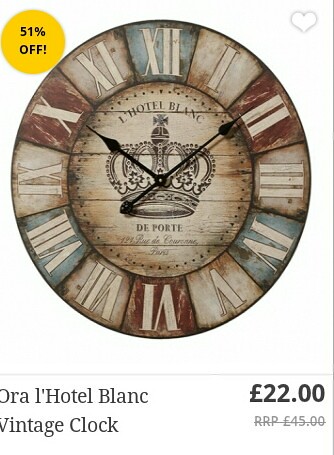The image is an advertisement for a vintage clock set against a pure white background. The clock, which resembles a rustic, modernized plate, features a circular design with alternating blue, tan, and brown sections for the hours, marked by white Roman numerals. The center of the clock displays a painted wood paneling backdrop with a distinct crown symbol where the black clock hands are positioned, indicating 10:10. Above the crown, the text "Le Hotel Blanc" is inscribed, and below it, "De Forte."

To the right of the clock, a vivid yellow circle with black text announces "51% OFF!" Above this circle is a faint gray-outlined heart icon, likely for a 'like' symbol. In the bottom-left corner of the image, a small white rectangle states "Oura Le Hotel Blanc Vintage Clock,” with a price tag of "22.00 pounds." This price is highlighted by the original price, "RRP £45.00," crossed out, emphasizing the significant discount.